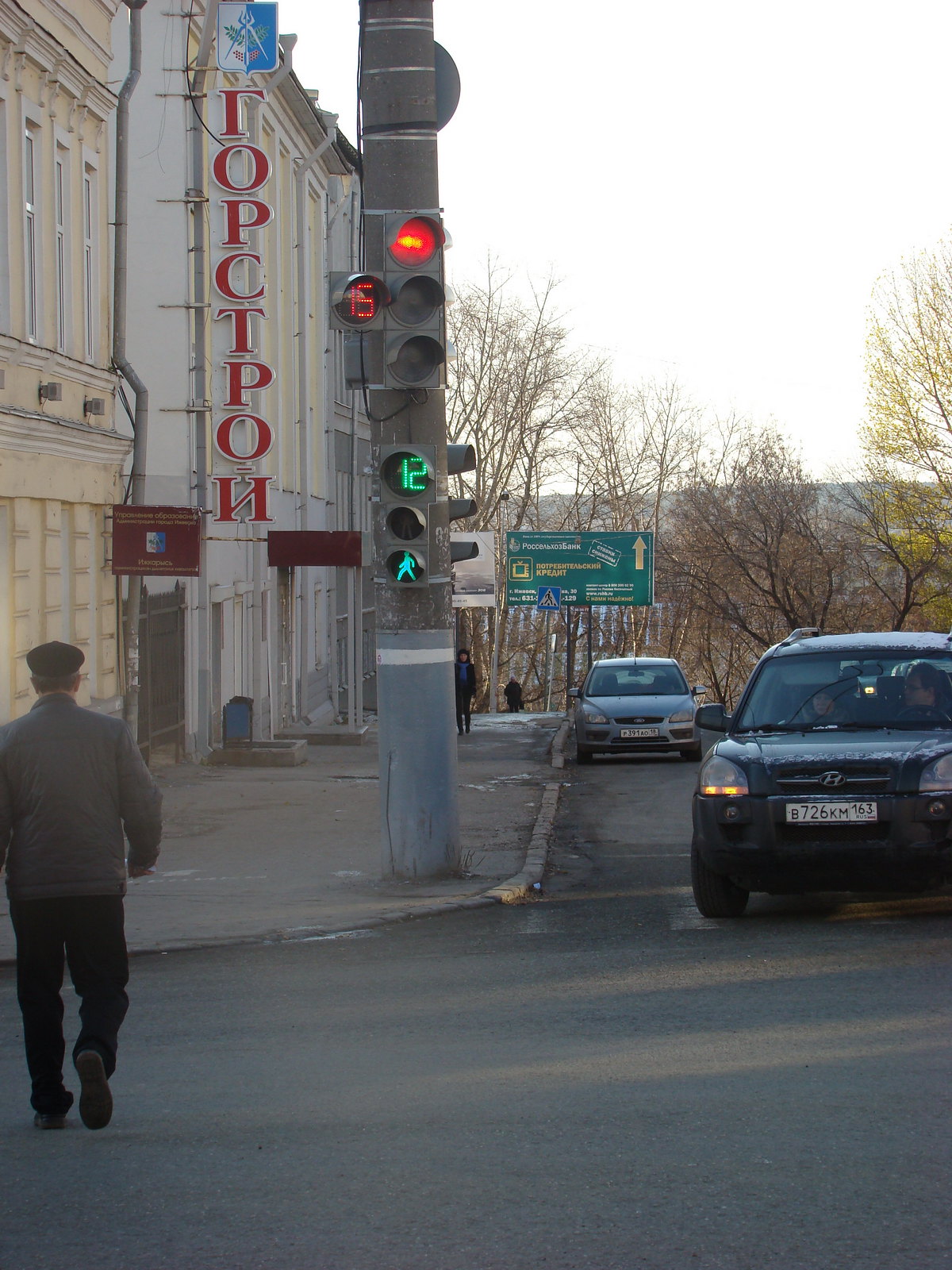This vibrant outdoor photograph captures a bustling intersection in a European city, possibly in Russia. A black Hyundai SUV with a white license plate reading B726 KM 163 R.U.S. is poised to make a right turn, while a man is crossing the street. The pedestrian signal glows green, indicating 12 seconds left for crossing. Simultaneously, a red light displays a countdown of 15 seconds for vehicles. The intersection is adorned with various traffic signs and signals, amidst a backdrop of rolling hills and sparse trees. Prominently, one building with Cyrillic writing that appears to spell РОСТРОЙ stands out, suggesting the Russian locale. There's also a parked Ford car visible. Additionally, a green street sign with a yellow arrow is noted in the background, contributing to the intricate details of this lively street scene.